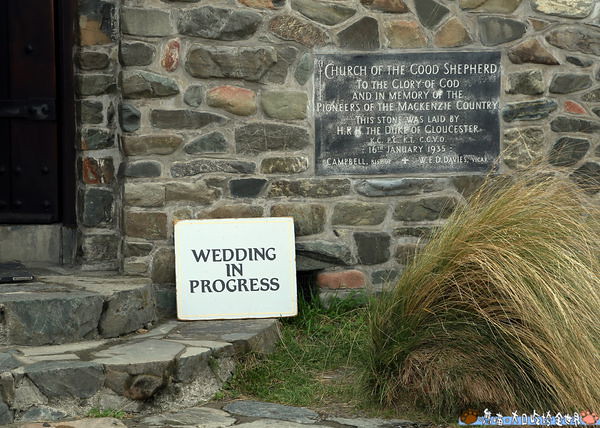This photograph captures the entrance of a historic church, the Church of the Good Shepherd, from an outdoor perspective. The scene prominently features the stone-clad facade of the church with its heavy, dark wooden entrance door partially visible on the left side of the image. Two stone steps lead up to the door, and on one of these steps sits a white sign with black letters that reads "Wedding in Progress." An engraved marble plaque on the stone wall bears the inscription: "Church of the Good Shepherd, to the glory of God, and in memory of the pioneers of the Mackenzie country. This stone was laid by His Royal Highness, the Duke of Gloucester, 16th January 1935." In the foreground, a pathway bordered by tall, beach grass-like shrubs leads up to the steps, enhancing the rustic and serene setting of this picturesque church entrance.